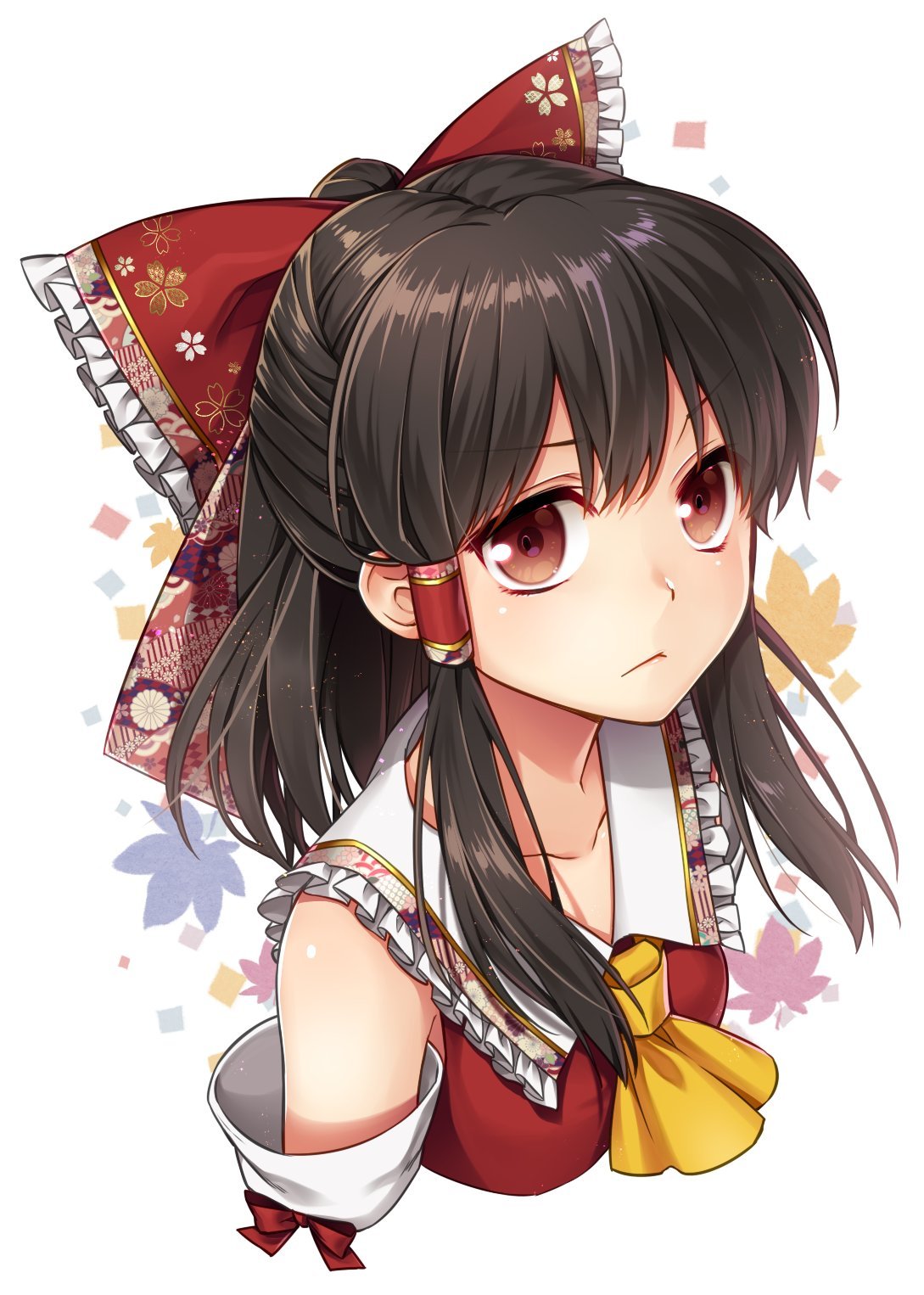This is an intricately detailed anime-style portrait of a young girl, likely around 8 to 10 years old, set against a white background with colorful confetti and leaves in shades of yellow, green, red, and purple gently falling around her. The girl has large, expressive hazel brown eyes, a small characteristic anime nose, and a subtle frown on her face, imparting a sense of sadness. Her medium brown hair is styled with bangs over her forehead, and longer sections on the sides are pulled back into a pigtail held by a cylindered wrap. 

A prominent red bow adorns the back of her head, featuring white fringing on the corners and intricate gold and white oriental-style floral patterns. The ribbons of the bow extend down with a white ruffle trim that resembles lace. She wears a red top with a white collar that forms a V-neck, trimmed in the same ruffled material as the bow. A yellow bow tie is knotted at the front center of her chest, adding to the overall aesthetic. Her outfit also includes a white sleeve with a red bow on the side, visible only from her shoulder down to her elbow. The colorful background elements and detailed clothing design emphasize the anime aesthetic while highlighting her melancholic expression.